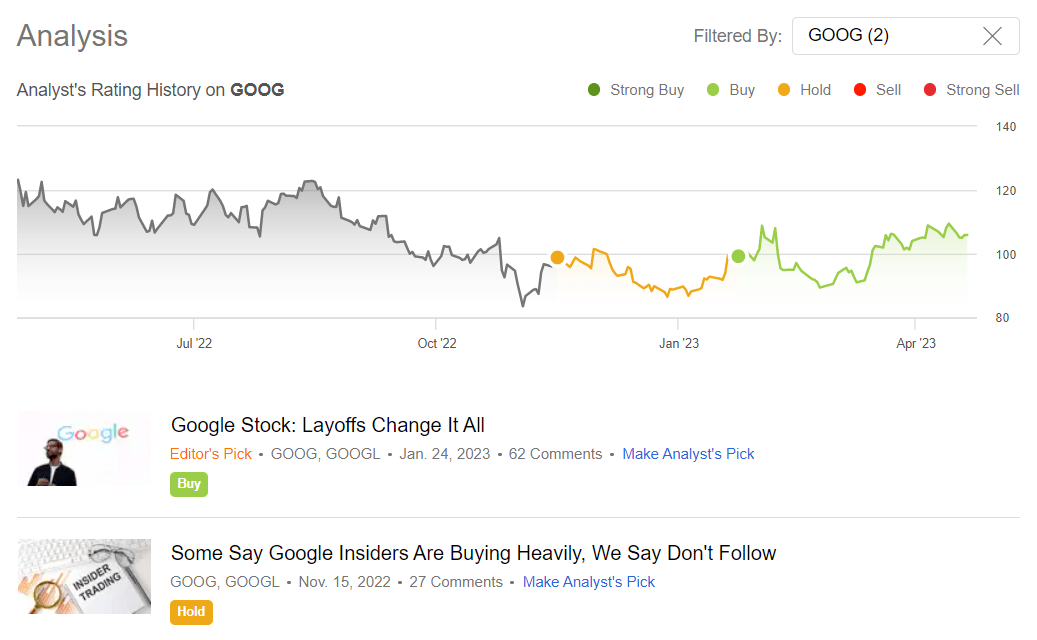A cropped screenshot from a webpage, focusing solely on a line graph, titled "Analysis" in grey text. This graph presents data spanning from July 2022 to April 2023, with the vertical axis scaled from 80 to 140. The graph is equipped with a legend featuring five color-coded categories: Strong Buy, Buy, Hold, Sell, and Strong Sell. The chart specifically analyzes GOOG, presumably Google Stocks, and visually depicts the fluctuations in their current rating over the specified period.